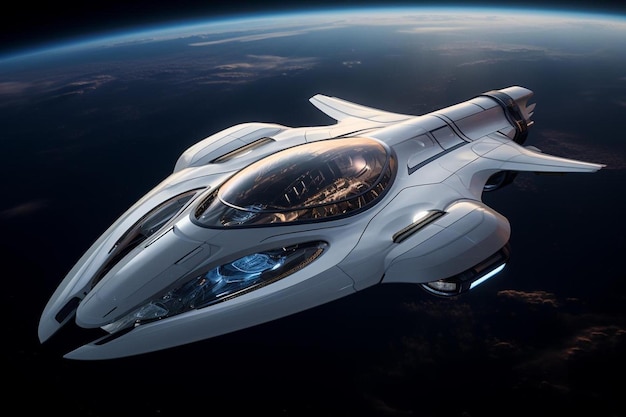The image depicts a highly detailed, futuristic spaceship, seemingly computer-generated or a meticulously crafted 3D model, floating above Earth. The spacecraft, resembling a blend between an advanced aircraft and a spaceship from a sci-fi film like Star Wars, features a sleek, off-white or gray body. It possesses wings at the back and a front design reminiscent of an F1 race car, with pointed ends.

Central to the spaceship is a transparent, amber-tinted cockpit, potentially accommodating one or two individuals. The design incorporates glass panels on either side of the front, allowing a view into the ship's engine, which emits a blue fluorescent glow, suggesting an ion or futuristic power source. The image is taken from a perspective that showcases Earth as a prominent, blue orb in the background, filling up most of the frame and accentuating the spaceship's small scale relative to the planet. Overall, the spaceship exudes a cutting-edge, futuristic appearance, enhanced by its contemporary and plane-like elements, and is set against the awe-inspiring backdrop of Earth's curvature.